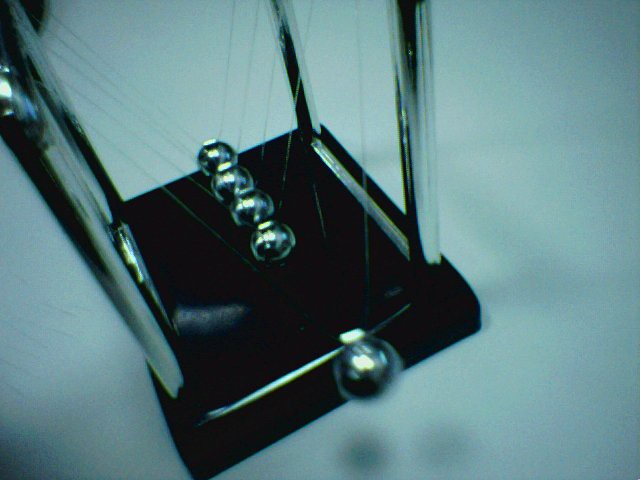This black-and-white photograph features the iconic Newton's Cradle, often referred to here as Einstein's Pendulum. The scene captures the device, typically found on many office desks, with its five shiny, metallic silver balls suspended by clear nylon strings. The balls, which operate on the principles of momentum and energy transfer, are elegantly lined up on a sleek black plastic base. The device includes four chrome-colored vertical supports placed on each corner, with matching horizontal bars connecting them at the bottom, giving it a sturdy frame. In the image, one ball is seen in motion, swung back and about to hit the remaining static balls, demonstrating the classic back-and-forth movement characteristic of the Newton's Cradle. Despite the setting being dark and the image somewhat blurry, the silver balls and their dynamic movement are clearly discernible, emphasizing the elegant simplicity and perpetual motion of this scientific toy.